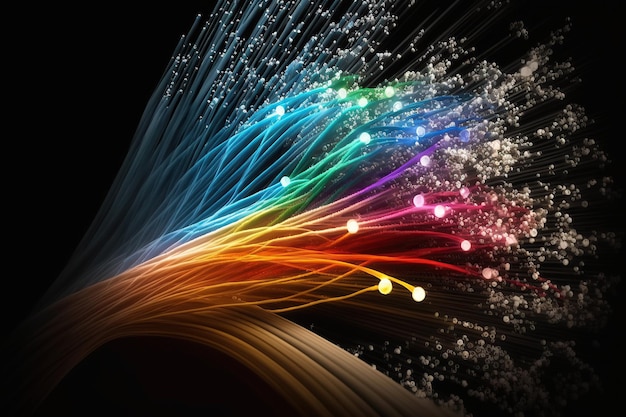The rectangular digital image, approximately four to five inches wide and three inches high, showcases a vivid, black background with an intricate array of radiant lines. These lines, extending from the lower left-hand corner across the image, represent a dazzling spectrum of colors including red, orange, yellow, green, turquoise, blue, purple, magenta, and more. Resembling an explosion of color or a vibrant firework display, the lines are intertwined and branching out like a tree. Many of these strands feature bright white circular shapes or small, shiny bulbs at their tips, giving the impression that the lines are glowing brightly in the dark. The multicolored lines, some appearing as painted cables, are intricately designed to highlight the vividness and blend of colors, conjuring a sense of dynamic movement and luminescence against the stark black background.